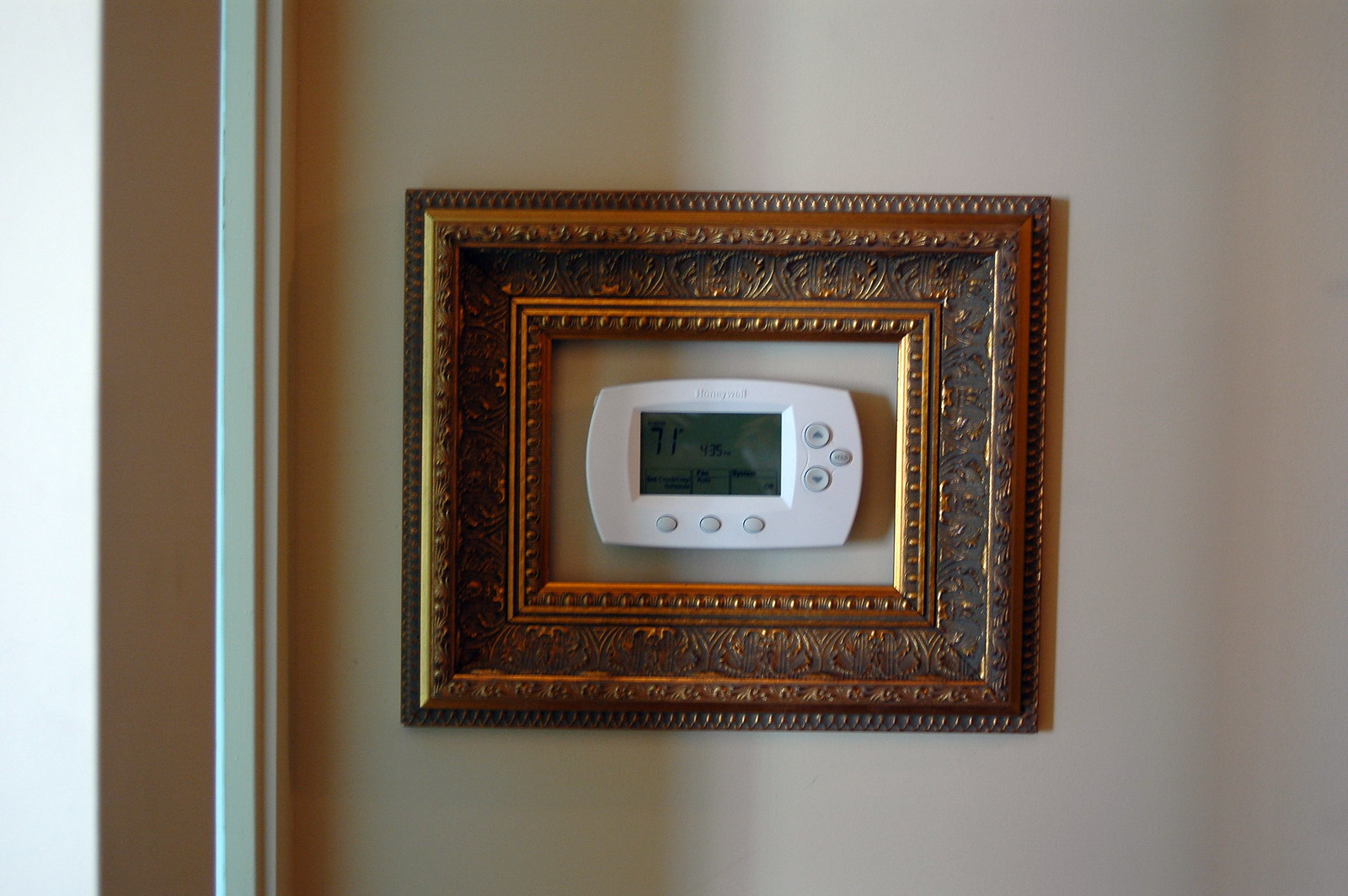The image features a thermostat prominently displayed on a smooth, light beige or gray wall. To the left, the wall is bordered by a door frame made of wood painted in white, suggesting the thermostat is located near a doorway. Adding an artistic touch, the thermostat is encased within a small, ornate picture frame, which is gold-colored with a textured pattern, giving it a decorative appearance. The thermostat itself is white and bears the branding "Honeywell," indicating its manufacturer. The device has six buttons for control surrounding a gray and black LCD screen. The screen displays crucial information, including the current temperature, which reads 71°F, and the time, showing 4:35 p.m.